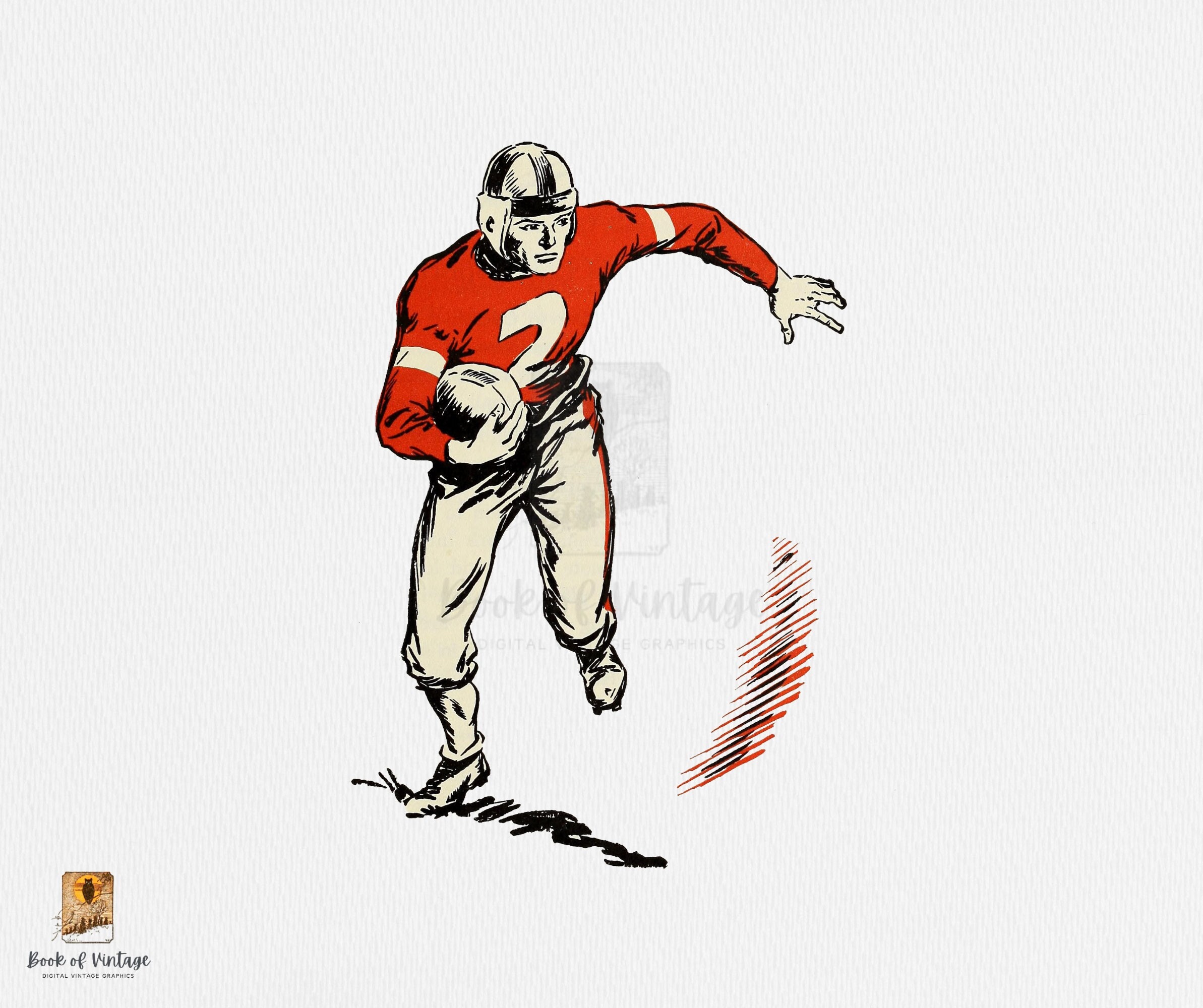This detailed colored pencil drawing, possibly from a vintage book, captures an early 1900s American football player in mid-run. The player has fair skin and dons a distinctive white leather helmet covering his ears. His red long-sleeved jersey features a striking white number 2 on the front and white bands around the biceps. Complementing his jersey, he wears beige football pants with a red stripe down the thigh and beige cleats designed for grip on the grass.

The athlete is seen dashing towards the viewer but looking to his left, with his right hand clutching a football and his left arm and leg dynamically positioned, conveying motion. Below his right foot, black squiggly lines suggest grass, enhancing the sense of movement.

In the lower left corner, the text "Book of Vintage" is elegantly inscribed in cursive, accompanied by a logo featuring an owl and a scene of horses ascending a hill towards the sun, rendered in brown, yellow, and white hues. A light watermark bearing this same icon overlays the image, adding to its vintage aesthetic. The setting and details vividly evoke the early days of American football, encapsulated in a charming, retro artistic style.